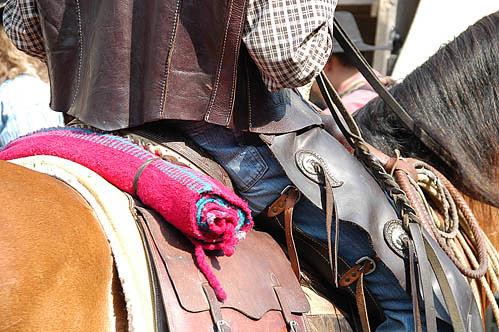In this richly detailed, close-up color photograph in landscape format, we see a segment of a Western rider atop a bay horse. The shot focuses on the area from the rider's elbows to their knees, capturing their attire and gear with clarity. The rider sports faded blue jeans, leather chaps, a brown leather vest, and a brown and white checkered shirt. In their right hand, they firmly hold the leather reins. The dark-maned bay horse is shown from just behind the saddle halfway up its neck, emphasizing its solid build. 

The Western-style saddle is adorned with various items: a coiled lariat hangs in front of the rider's leg, a brown saddlebag sits behind the rider's knee, and a distinctively pink and blue rolled-up Indian blanket is fastened behind the cantle. The scene is full of subtle elements, such as other figures in the background—a woman with blonde hair and a blue sweater and a man in similar Western attire, including a cowboy hat—though they remain mostly out of focus. The resulting image captures the essence of Western riding with meticulous attention to detail in both attire and gear.